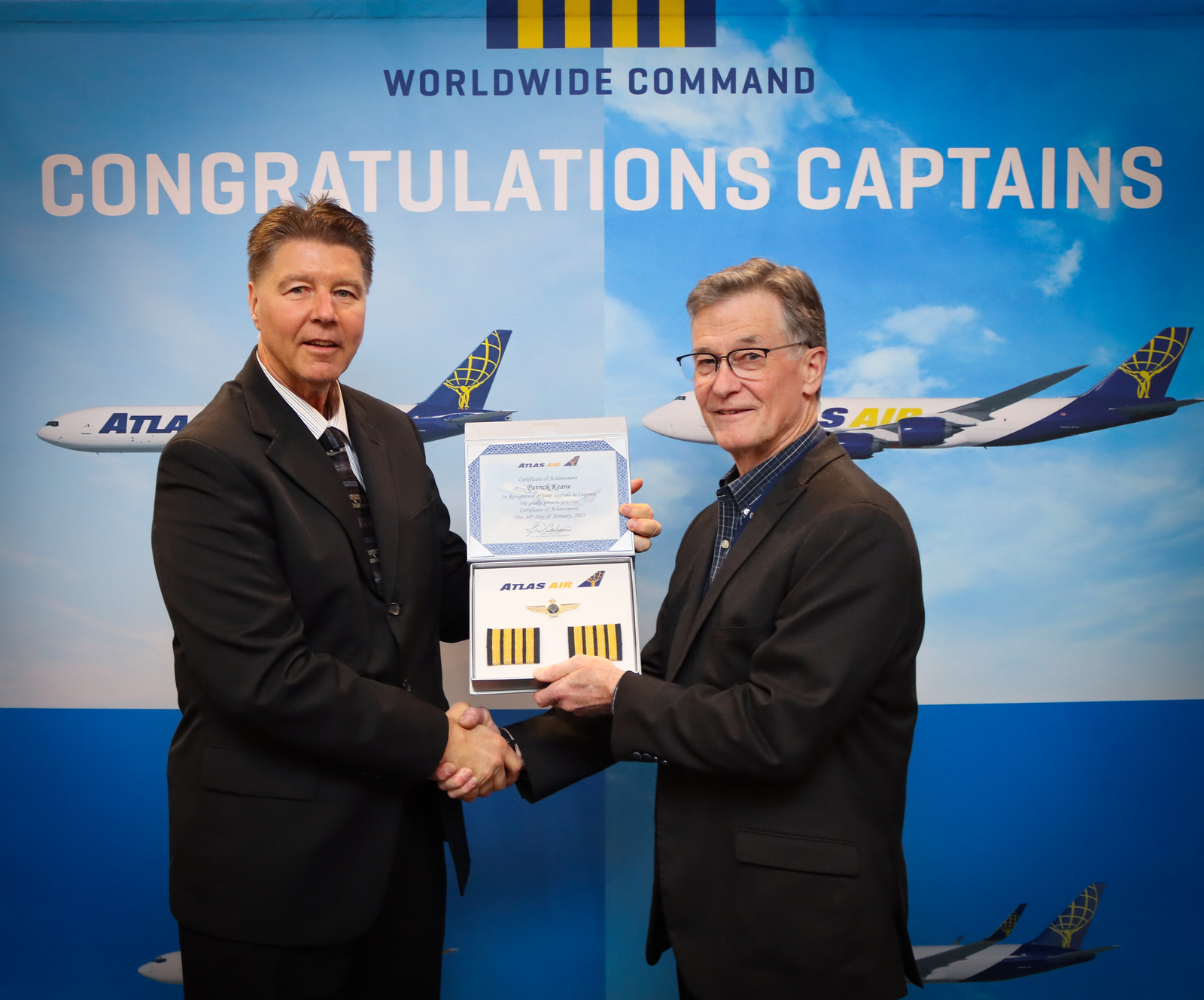Two men stand facing each other, shaking hands with their right hands while each rests their left hand on an award inscribed with "Atlas Air." This award features two squares near the bottom, each adorned with four vertical gold stripes. The man on the right, who wears glasses and has a dark suit jacket over a blue and white plaid shirt, looks directly into the camera. The taller man on the left is dressed in a dark suit, white shirt, and tie. Behind them, a backdrop displays the words "Congratulations, Captains" in white lettering, along with the phrase "Worldwide Command." The background is also decorated with images of two airplanes, symbolizing their achievement in aviation.